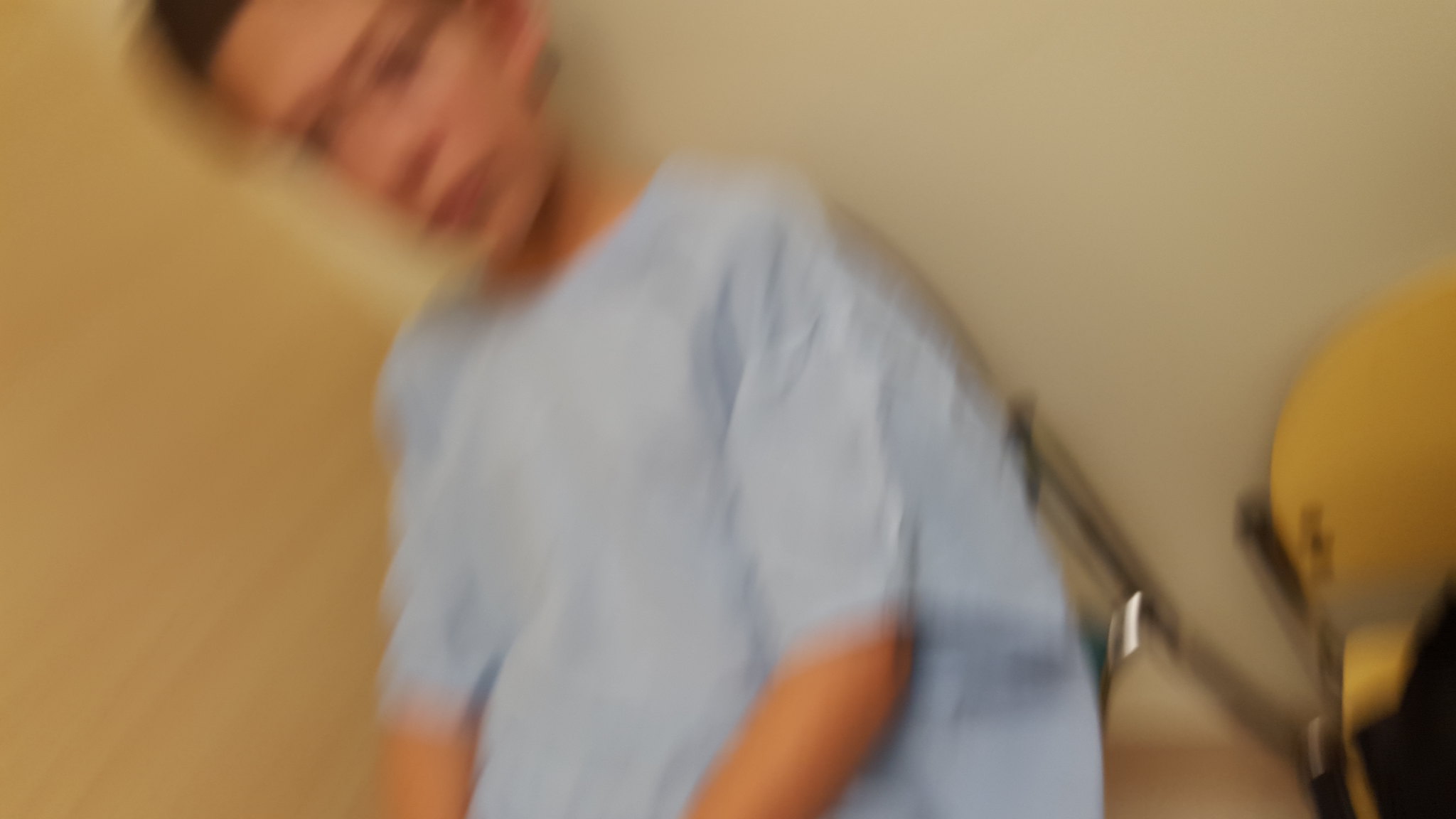This is a blurry, somewhat skewed photograph taken indoors, capturing a young Caucasian boy, estimated to be between 12 to 15 years old, sitting on a chair with a chrome frame. He has short, dark brown hair, dark eyebrows, and brown eyes, and his expression appears sad, with his head slightly tilted to the left. He is wearing a very loose, light blue shirt that resembles a hospital gown. The background features a wall that is a mix of dark beige and light tan. To the right of the boy is another chair, characterized by a light wooden back and chrome frame. Overall, the entire scene, including the furniture and wall, is out of focus, giving the image a hazy, indistinct quality.